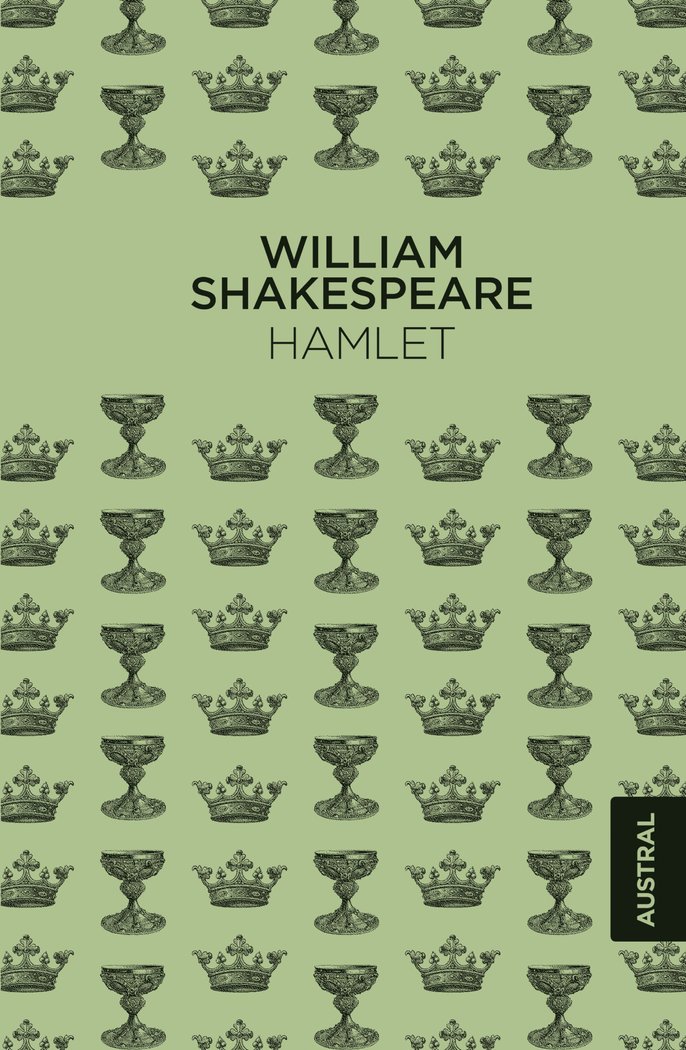The image appears to be the cover of a playbook for William Shakespeare's *Hamlet*. The background is a light sage green color with a repeating pattern of black crowns and chalices arranged in vertical rows. The crowns feature a tall point in the center flanked by smaller and taller outward-bending points, while the chalices have a wide cup top and circular base. About one-third down from the top, there is a blank space where "William Shakespeare" is written in bold black capital letters, with "Hamlet" below it in non-bold capital letters. Towards the bottom right corner, there is a small black box containing the word "Austral" in a matching green font, indicating the publisher.